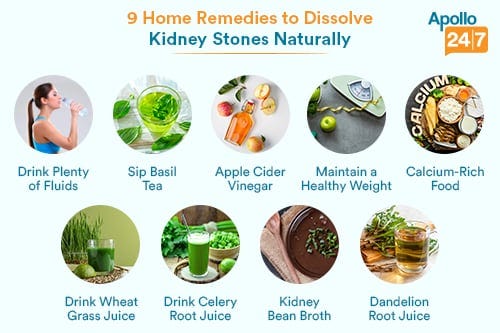This infographic, set against a light blue background, presents "9 Home Remedies to Dissolve Kidney Stones Naturally" as detailed in yellow and green text at the top. The top right corner features the Apollo 24/7 logo. The visual guide is split into two rows of images, each accompanied by text descriptions.

In the top row:
1. A woman with a brown ponytail drinks from a water bottle, highlighting the remedy "Drink plenty of fluids."
2. A cup of basil leaves with the caption "Sip basil tea."
3. Apples and a glass jar of light brown liquid next to "Apple cider vinegar."
4. An apple, a tape measure, and a scale, indicating "Maintain a healthy weight."
5. Various cheeses with the tag "Calcium-rich foods."

In the bottom row:
1. A glass of green liquid labeled "Drink wheatgrass juice."
2. A taller glass of green liquid marked "Drink celery root juice."
3. A bowl of brown liquid with a wooden spoon captioned "Kidney bean broth."
4. A glass of clear brownish liquid annotated "Dandelion root juice."

Each image serves as a visual aid to represent the natural remedy suggested, enhancing the infographic’s informative and accessible approach.